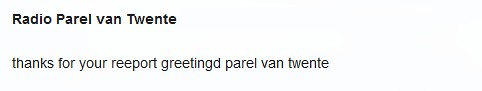The image features a sparse, horizontally aligned rectangular banner with a very faint blue background. Positioned at the top right, the text in a mix of upper and lowercase letters reads "Radio Parallel of on 20". A few lines beneath, in smaller and fainter print, the text "thanks for your report, greeting the peril of on Twente" appears. Notably, the words are riddled with typos: "thanks" starts with a lowercase 't', "report" is spelled "reeport", and "greeting" is spelled "greetingd". The overall style suggests a European influence, possibly by someone prone to making frequent typographical errors. The text is black, and there are no other features or borders in the image.